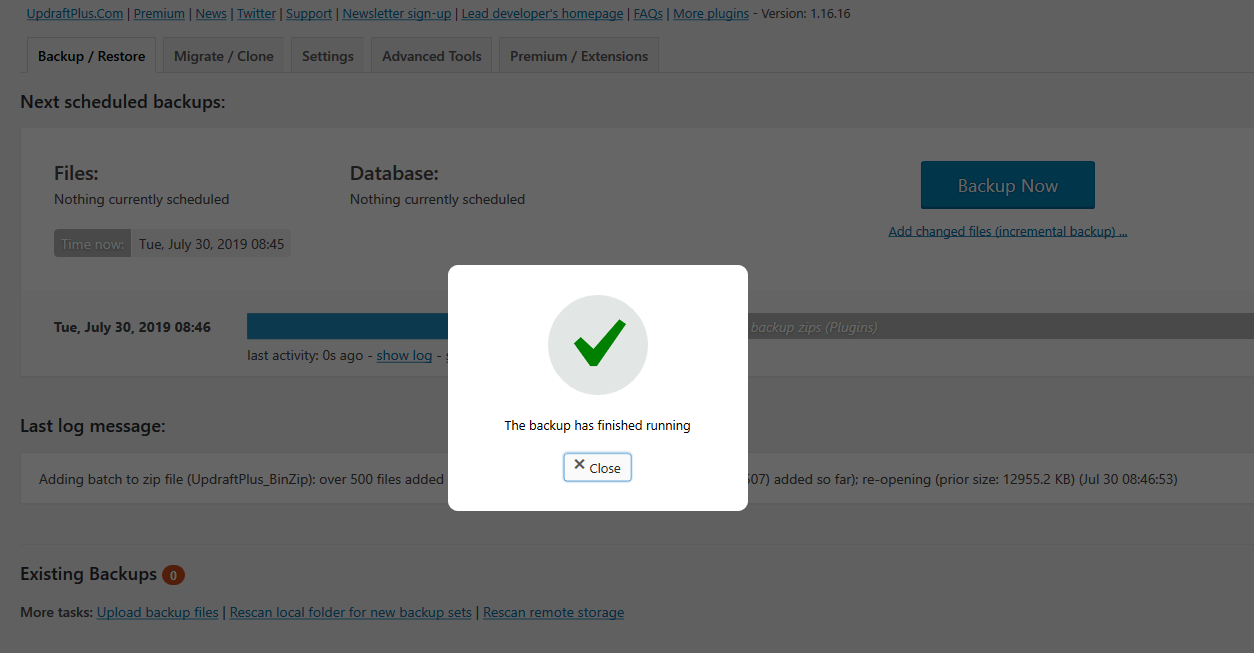The screenshot displays the user interface of the UpdraftPlus backup plugin for WordPress. At the top of the interface, there is a navigation menu with various options, all of which are hyperlinked and displayed in blue. The options include "updraftplus.com," "premium news," "Twitter," "support," "newsletter sign up," "Lead developers homepage," "FAQs," "more plugins."

Below the navigation menu, there are several tabs, with the current one being "Backup/Restore." Other available tabs include "Migrate/Clone," "Settings," "Advanced Tools," and "Premium Extensions." 

In the "Backup/Restore" tab, the section titled "Next scheduled backups" is displayed in black text. Beneath this heading, a long horizontal white box contains information about scheduled backups. Currently, there are no scheduled backups for files or the database, which is indicated by the text "nothing currently scheduled." The current date and time are displayed as "Tuesday, July 30, 2019, 8:45."

To the right of this information, there is a large blue "Backup Now" button and an "Add/Change Files" hyperlink. Additionally, a notification box with a checkmark indicates that a backup has completed, accompanied by a "Close" button.

Returning to the white horizontal box, it further reiterates the current date as "Tuesday, July 30th," and shows a partly filled progress bar for the backup zip file. An adjacent log message indicates "adding to zip files UpdraftPlus," along with the note "existing backups currently shows zero."

The interface also includes three blue hyperlinks: "Rescan local folder for new backups," "Rescan remote storage," and "more tasks that pull back files."